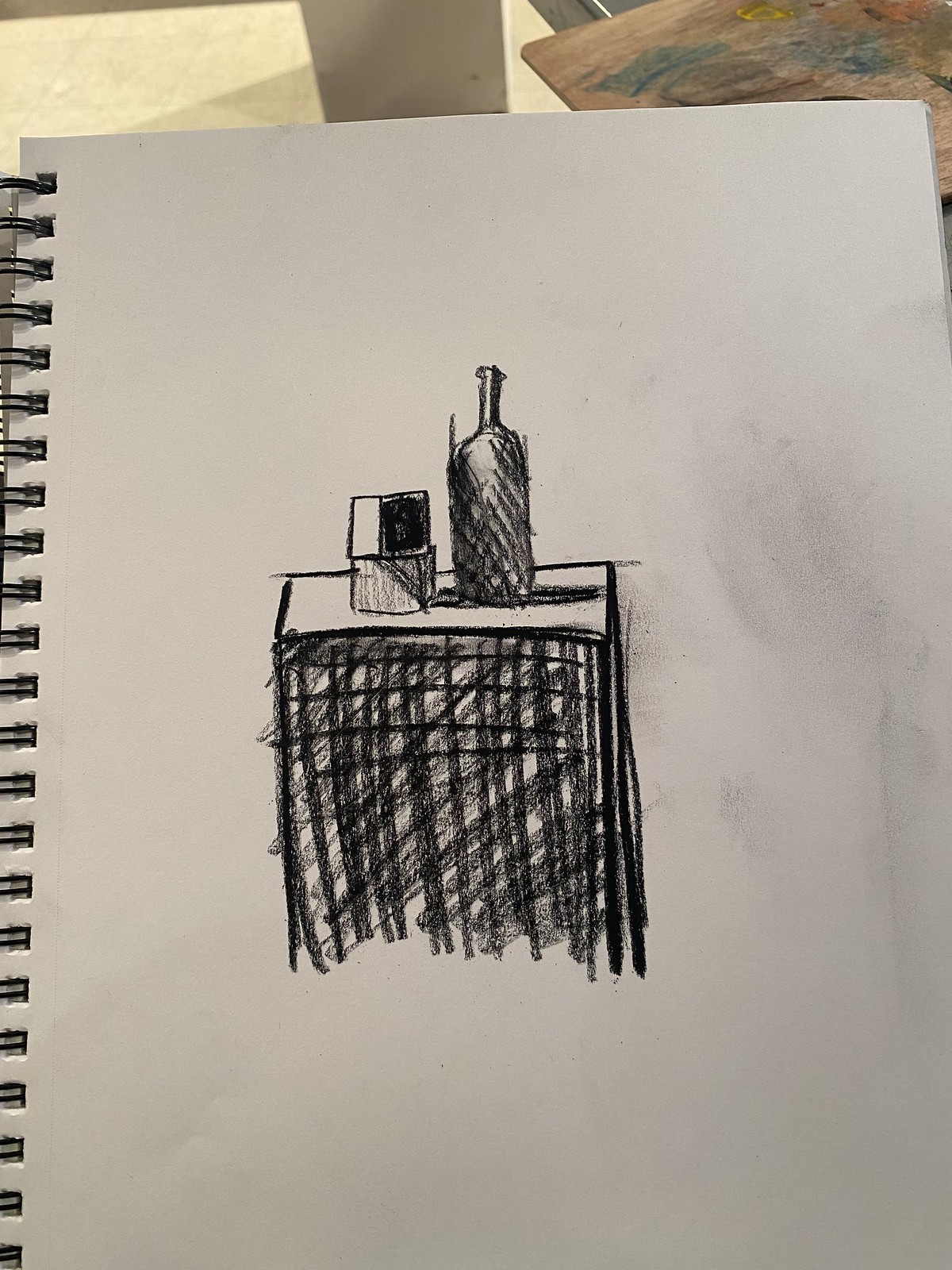This photograph captures a spiral-bound sketchbook resting on a white table, surrounded by indistinct objects. The sketchbook, featuring black wire spirals and pristine white pages, is open to reveal a detailed drawing. The artwork depicts a table adorned with two bottles. The table's surface is white, while its legs are drawn with black diagonal lines, accentuated by vertical and horizontal strokes to create a sense of depth and texture.

The bottle on the left is shorter, appearing transparent with meticulous shading to convey its cylindrical shape. Its screw-off lid is darker on one side, suggesting a light source. The taller bottle on the right mimics the form of a slender vase or liquor bottle, distinguished by a narrow neck and a crosshatch design that adds dimensionality. Both bottles cast shadows on the table, enhancing the realism of the scene.

A noticeable smudge to the right of the drawing suggests possible interaction with the artist's hand, hinting at the use of charcoal as the medium, which might have transferred to the paper inadvertently.